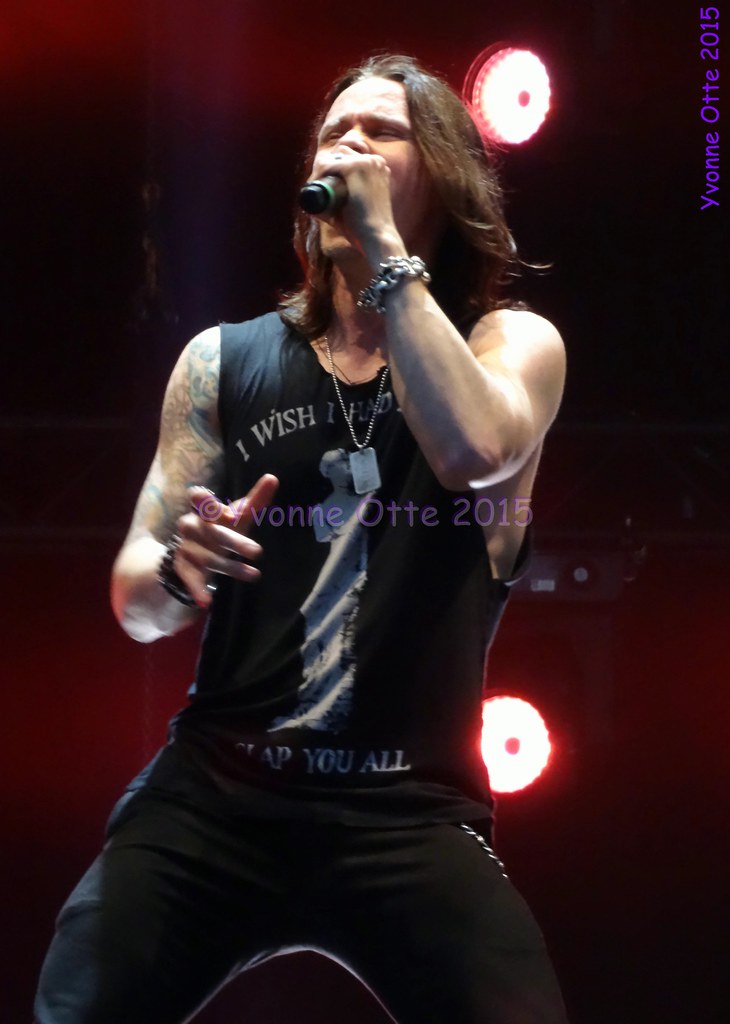The professionally shot photograph captures a dynamic moment from a concert, focusing on a rock singer with long, shoulder-length brown hair. He is energetically singing into a microphone held close to his face, obscuring most of his facial features. He sports a sleeveless black tank top adorned with a white Michelangelo statue graphic, partially obscured by his arm, and purple accents, which have visible white lettering. His attire includes black jeans and accessories like black beads on his right wrist, silver beads on his left wrist, and a silver chain necklace with a dog tag. The singer's right arm features a tattoo sleeve extending from his shoulder to his elbow. The low-angle shot, which adds a sense of grandeur, also captures red lighting behind him that creates a striking black and reddish backdrop. The upper right corner of the photograph includes the photographer's watermark, "Ivan Ott 2015," and the scene is set indoors, suggested by the scaffolding supporting the lights.